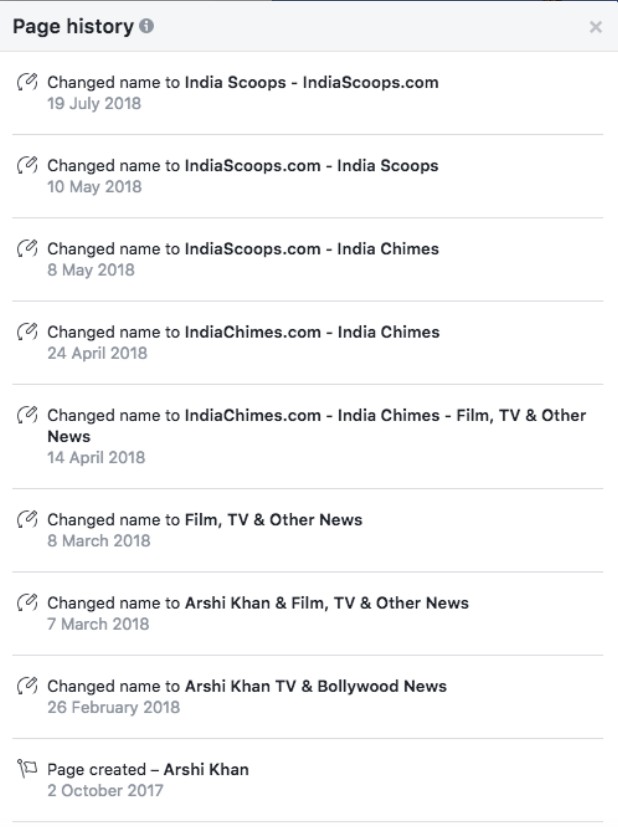The image depicts a screenshot of a page history section, which could be from a website or an app. The overall design utilizes light colors with black text. At the top, a light gray bar stretches across the width of the page. On the left side of this bar, "Page history" is displayed in black bold letters, with only the "P" capitalized. Adjacent to this text is an information icon, followed by a space, and then an "X" icon in gray located at the far right. 

A thin black border runs above the gray bar, while a light gray border of similar thinness lies below it. The primary content of the page is the history records. Within this section, there are approximately eight to ten rows detailing historical changes. 

Each row features an icon on the left, depicting a pencil inside a circular arrow, symbolizing edits. To the right of the icon is a bold text indicating the change, such as "Change name to indiascoops-indiascoops.com." Below this text is a timestamp, for example, "19 July 2018." Each row is separated by a thin gray line.

The last row differs from the rest; instead of the pencil icon, it displays a flag icon. The text next to it reads "Page created - arshi con," with a timestamp of "2 October 2017" below it, followed by a separating gray line. The entire layout is set against a white background.